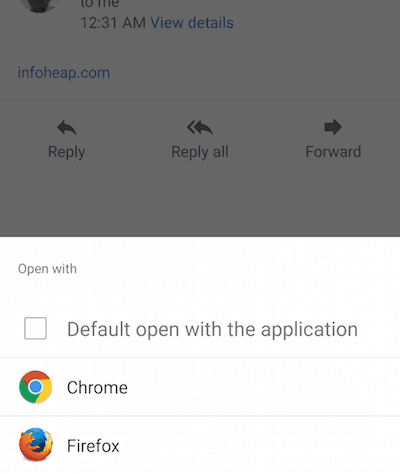The image depicts a computer interface focused on a pop-up window overlaying an email application. The background displays the top and bottom sections of an email composition page, including the "Reply," "Reply All," and "Forward" buttons, as well as the email recipient's address with user icons, indicating interactions with an email from InfoHeap.com.

In the foreground, a white pop-up window titled "Open With" appears, featuring two browser options: Chrome and Firefox. At the top of the pop-up, there is a checkable box next to the text "Default Open With Application," allowing users to set their preferred browser for opening links by default. Both browser icons are displayed with accompanying text in a straightforward black and blue font. The overall design of the pop-up is minimalistic, with white and grey tones dominating the color scheme, ensuring clarity and ease of use.